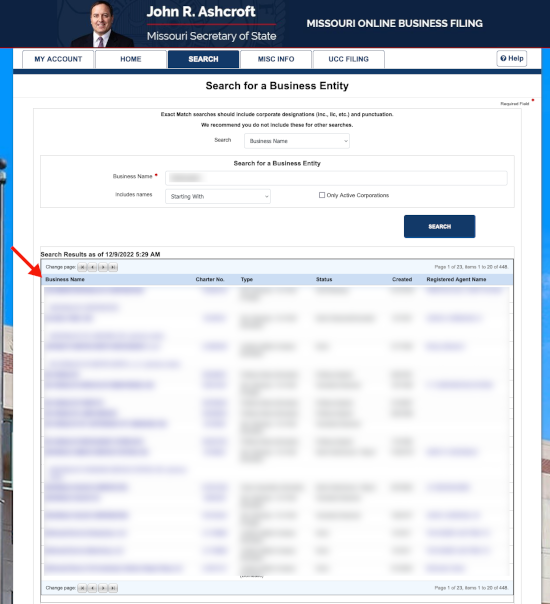The top of the page features a dark blue banner with a prominent layout. On the left side of this banner, an image of a man named John R. Ashcroft is displayed. This is identified by the text "John R. Ashcroft" written in white to the right of the image. Below this text, a red line acts as a divider. Underneath the red divider, written in a smaller, non-bold, white sans serif font, are the words "Missouri Secretary of State."

To the right side of the dark blue banner, the phrase "Missouri Online Business Filing" is displayed in bold, uppercase white lettering. Below the banner, there is a white toolbar that contains several menu options, all bordered in blue and written in bold uppercase blue font.

The menu options include:

1. "My Account" on the far left.
2. "Home" just to the right of "My Account."
3. "Search," which is the selected option, distinguished by a dark blue background with bold uppercase white font.
4. "MISC Info" next to "Search."
5. "UCC Filing" on the far right of the options.

On the extreme right end of the toolbar, there is a small rectangular icon with a blue border. Within the icon is a circular filled-in blue icon featuring a white question mark, accompanied by the word "Help" in blue.

Below the toolbar is a dark blue border transitioning into a white background. The header "Search for a Business Entity" is prominently displayed in bold black font.